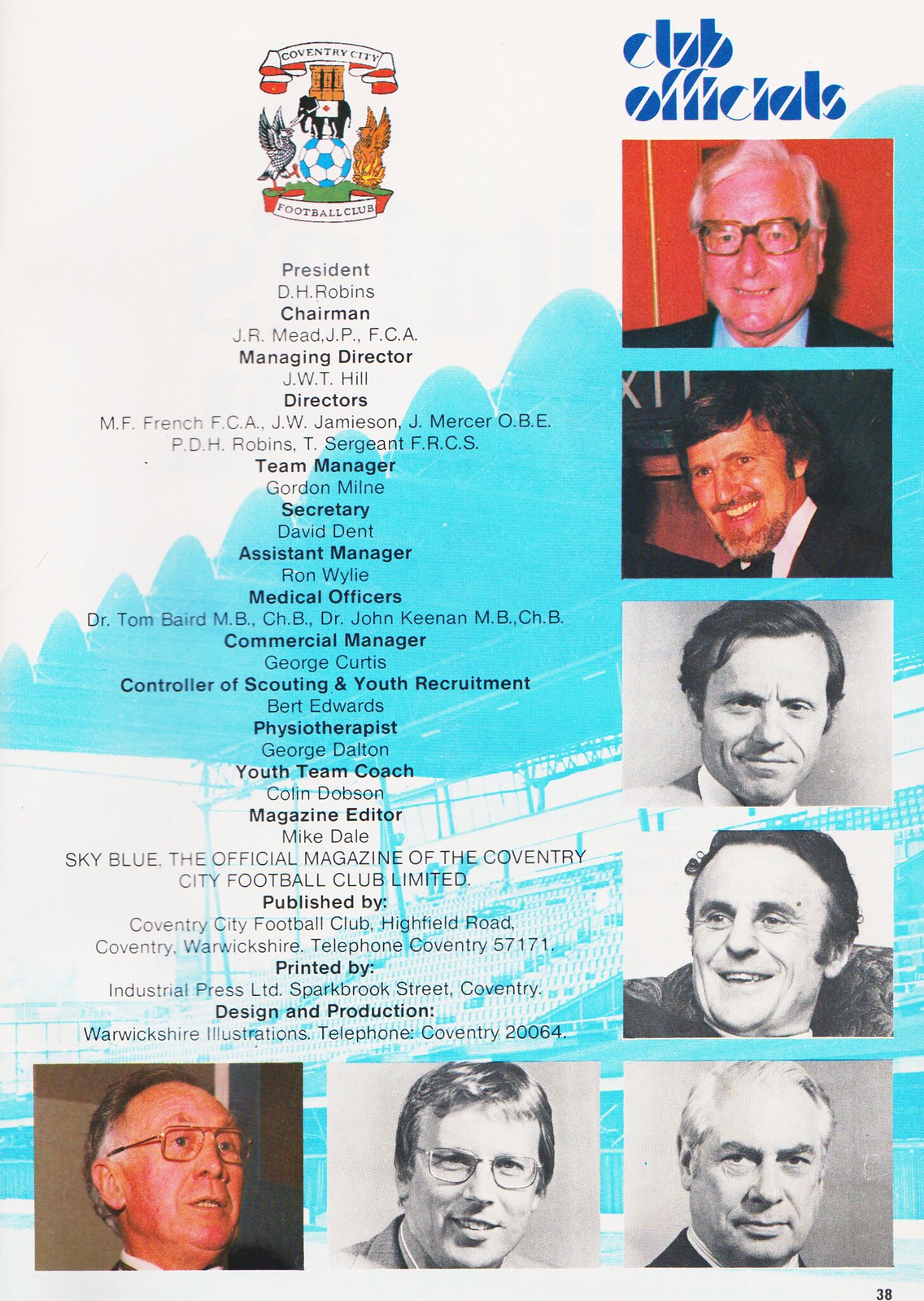The image is a detailed page from a Coventry City Football Club publication, possibly a yearbook or program. The background features a blue and white silhouette related to soccer, slightly obscured by the overlaid text and images. Prominently, in the upper right corner, the phrase "Club Officials" is displayed in blue font with white lines bisecting each letter. 

The top left corner is adorned with the colorful Coventry City Football Club crest, which includes a blue and white soccer ball flanked by what appear to be two dragons or eagles, with a white and red banner that reads "Coventry City" at the top and another at the bottom that says "Football Club."

Running from the top right corner downward and then extending to the left, the page features seven portrait photographs of male club officials. The arrangement of the photos forms a backward L shape, with three in color and four in black and white.

To the left of the photographs, the page lists details in black font about each of the officials, including their names and roles such as president D.H. Robbins, chairman, managing director, directors, team manager, secretary, assistant manager, medical officers, commercial manager, controller of scouting and youth recruitment, physiotherapist, youth team coach, magazine editor, and those responsible for publishing, printing, and design and production.

The page's number, 38, is noted at the bottom right, suggesting it is part of a larger magazine or book.